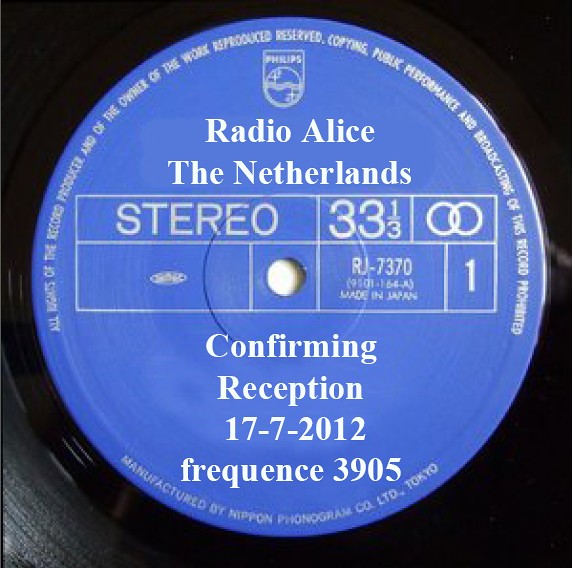The square photograph captures a close-up view of a vinyl record's center label. The record itself is black with a distinctive blue circular sticker at its core, almost touching the edges of the image frame. At the top of this blue label, in bold white font, it prominently reads "Radio Alice, The Netherlands." Just below, a wide white rectangle houses the text "STEREO 33 1/3," flanked by two overlapping circles, reminiscent of a Venn diagram. Further down, bold white letters state, "CONFIRMING RECEPTION 17-7-2012 FREQUENCY 3905." Encircling the bottom half of the sticker, small white text declares, "manufactured by Nippon Phonograph Co., Limited Tokyo." The label also mentions "made in Japan" and "RJ 7370." Additionally, there's a visible logo at the top identifying "Philips", and the perimeter of the label includes the phrase, "all rights of the record producer and the owner of the work reproduced, reserved copy in public performance broadcasting of this record prohibited."